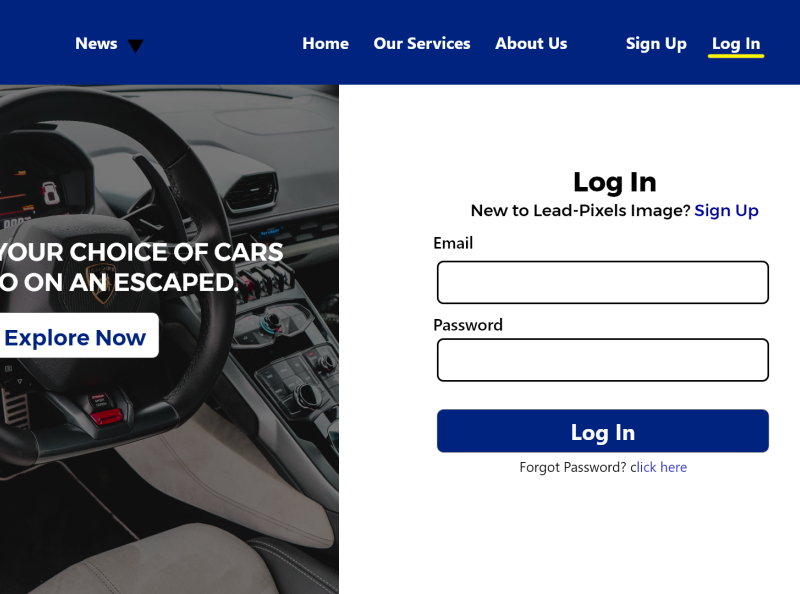A screenshot of a website's login page is presented without showing the web address bar. The page features a blue navigational bar at the top, containing options such as "News" with a dropdown menu arrow, followed by "Home," "Our Services," and "About Us." Further along the bar, options for "Sign Up" and "Log In" are displayed, with "Log In" highlighted by a yellow underline.

On the left side, there is an image depicting the interior of a car, specifically showing a steering wheel, gear shift, and part of the dashboard, with the text "Your Choice of Cars" partially obscured, displaying "O, O, On and Escaped." Below the text, a white button is labeled "Explore Now."

To the right, the login section invites users with "Log In," and for new users, "New to Lead-Pixels image? Sign Up." Below this, there are fields to enter an email address and password, accompanied by a large blue "Log In" button. A "Forgot Password" link is available for those who need it.

The background image to the left features a slightly hazy, futuristic vehicle interior, with its dashboard appearing mounted centrally, akin to where a cup holder might usually be, presenting a unique layout not seen in conventional vehicles. The strange textual elements "Your Choice of Cars, O, O, On and Escaped" suggest possible issues with the displayed content.